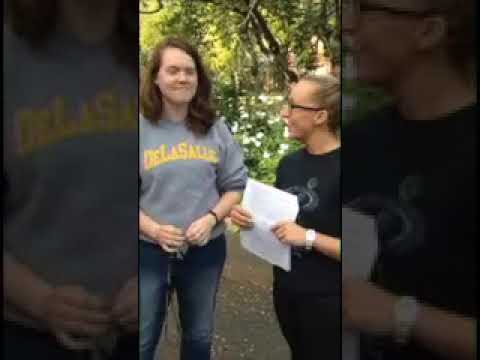In this very blurry, portrait-oriented outdoor image, two individuals stand amidst a backdrop of dense, leafy vegetation and twisting branches. On the left is a young white woman, possibly in her 20s, with shoulder-length brunette hair. She wears a gray sweatshirt featuring yellow lettering and a pair of blue jeans, her hands loosely together in front of her as she looks directly at the camera. To her right, partially cut off by the frame, is a white man wearing a black t-shirt and holding a piece of white printer paper. His glasses are faintly visible. The lower part of the image reveals a flat, brownish ground, likely cement or hard dirt, while thick black borders frame the sides of the picture.